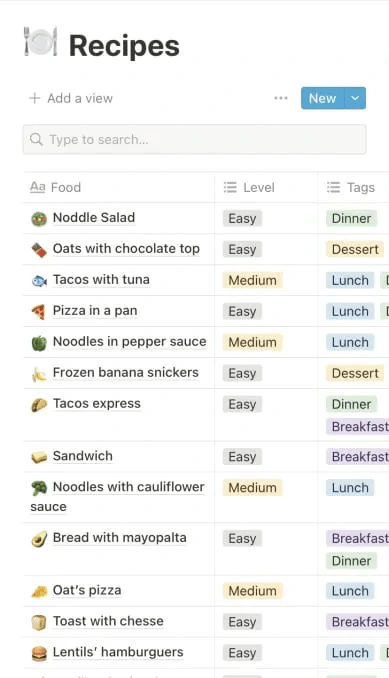This is a screenshot from a recipe website featuring a clean, predominantly white background. In the upper left corner, the website's logo is displayed: a white dinner plate with a fork on the left side and a knife on the right side. Next to this logo, the title "Recipes" is prominently shown.

Below the title, a blue "New" button with a drop-down menu is situated, accompanied by an "Add View" option with a small plus sign on its left. Directly below these, a search box is centered, currently empty.

The main body of the website is organized into three vertical columns: Food, Level, and Tags. Each row lists a recipe with its corresponding difficulty level categorized as easy, medium, or hard, and tagged meal type.

The recipes listed include:

1. Noodle Salad (Easy, Dinner)
2. Oats with Chocolate Top (Easy, Dessert)
3. Tacos with Tuna (Medium, Lunch)
4. Pizza in a Pan (Easy, Lunch)
5. Noodles and Pepper Sauce (Medium, Lunch)
6. Frozen Banana Stickers (Easy, Dessert)
7. Taco Express (Easy, Dinner)
8. Sandwich (Easy, Lunch)
9. Noodles with Cauliflower Sauce (Medium, Lunch)
10. Bread with Mayo Palta (Easy, Breakfast)
11. Oats Pizza (Medium, Breakfast)
12. Toast with Cheese (Easy, Breakfast)
13. Lentils Hamburger (Easy, Lunch)

The tags column classifies the recipes further into meals like Dinner, Dessert, Lunch, and Breakfast, providing users with an organized and easy-to-navigate overview of recipe options based on their meal preferences.